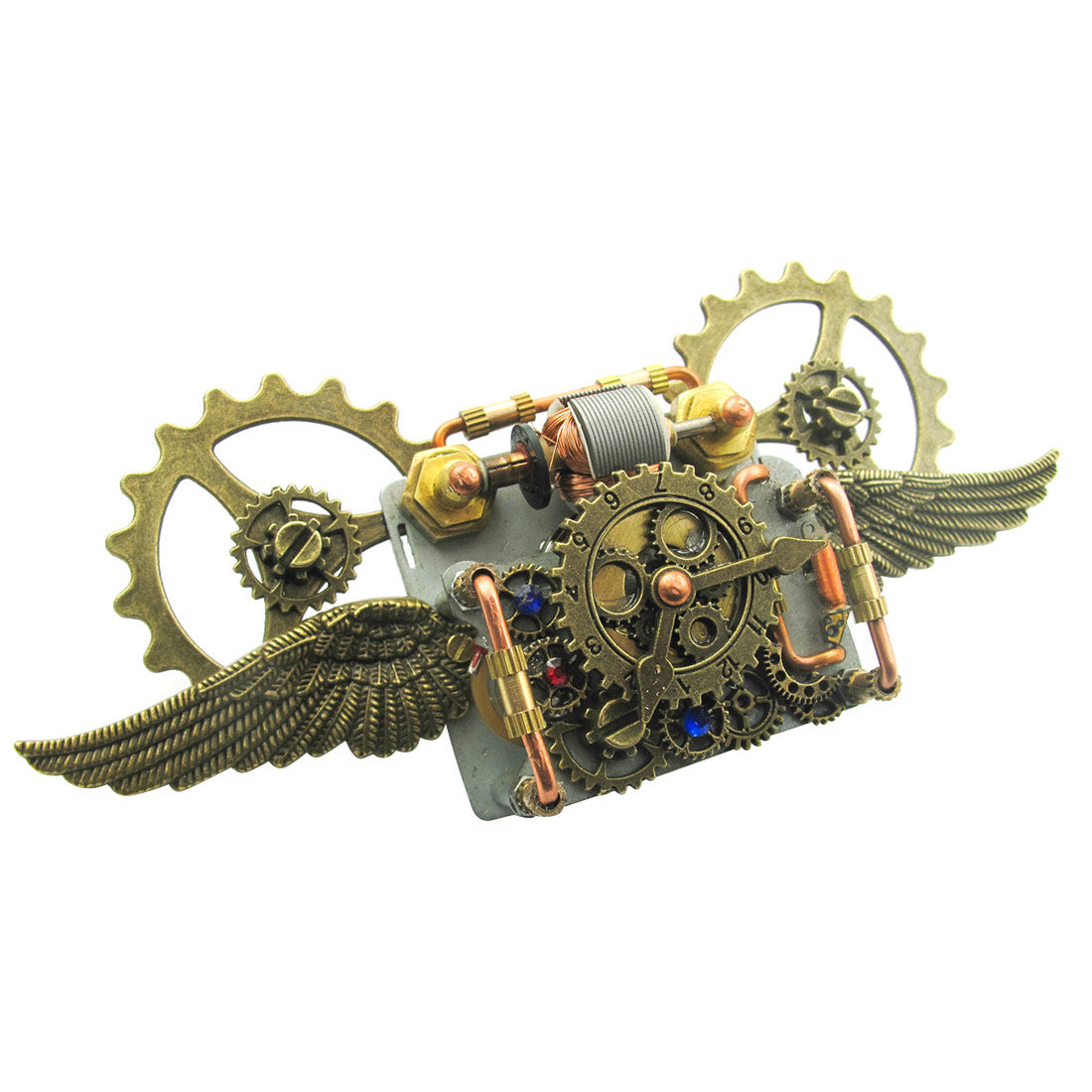The image depicts a bizarre, photorealistic mechanical contraption set against a solid white background. Central to the device is an upside-down clock face, tilted slightly to the right so that the 12 is near the 6 but shifted a bit. The clock has two hands of differing lengths, with the longer hand extending further across the face than the shorter one. Surrounding the clock face are various mechanical features: on either side are bronze or gold wings with intricate feather patterns, and in the upper left and right corners are large cog wheels also made of gold. Below the clock face and towards the left, there are several smaller, colorful cogs, each distinctly marked—one is a dull blue, another a ruby red, a third has a light sapphire hue, and a fourth has another cog overlaying it. Additionally, copper or bronze handles extend from either side of the clock face, adding to the complex structure of the device, which appears angled as if in flight. All these elements combine to create a detailed and intricate mechanical design that is both surreal and captivating.